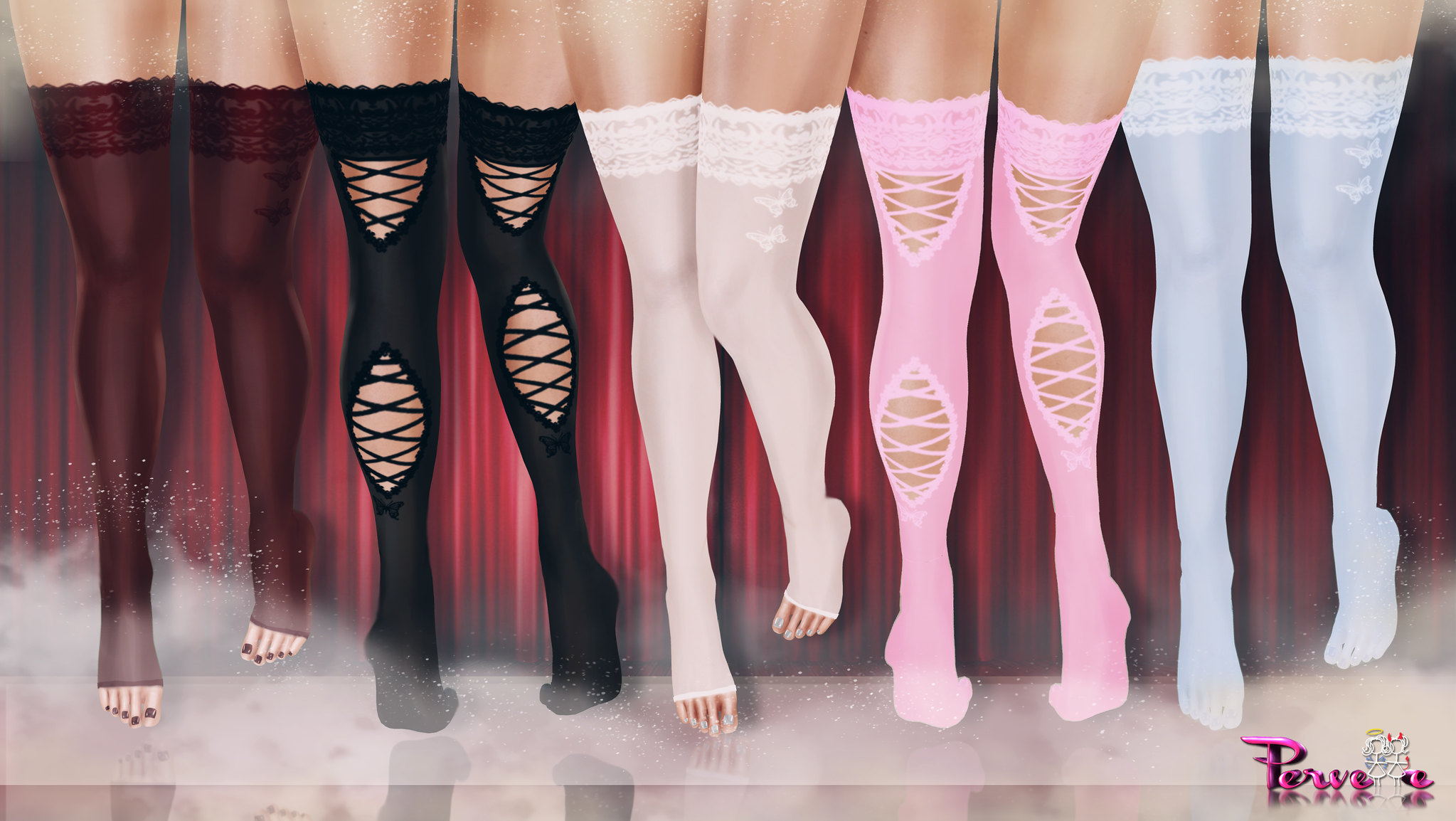This advertisement showcases a collection of thigh-high stockings and pantyhose in various styles, patterns, and colors. The image features five sets of legs, some facing forward and some backward, displaying the diversity of the stockings. On the far left, there are solid brown, toe-less stockings. Next, there are ones with a fishnet design around the knee and calf, these having closed toes. There's also a set of all-white, open-toe stockings adorned with delicate lace butterfly embroidery. Another pair, also depicting the back view, mirrors the fishnet design but with closed toes. Lastly, solid white stockings feature the same butterfly embroidery but with closed toes. The bottom right corner contains a partially legible logo, possibly "P-E-R" or "P-E-W-E," suggesting the brand. Each pair reflects different designs, including sheer fabric, lace, and intricate patterns, catering to a variety of preferences.